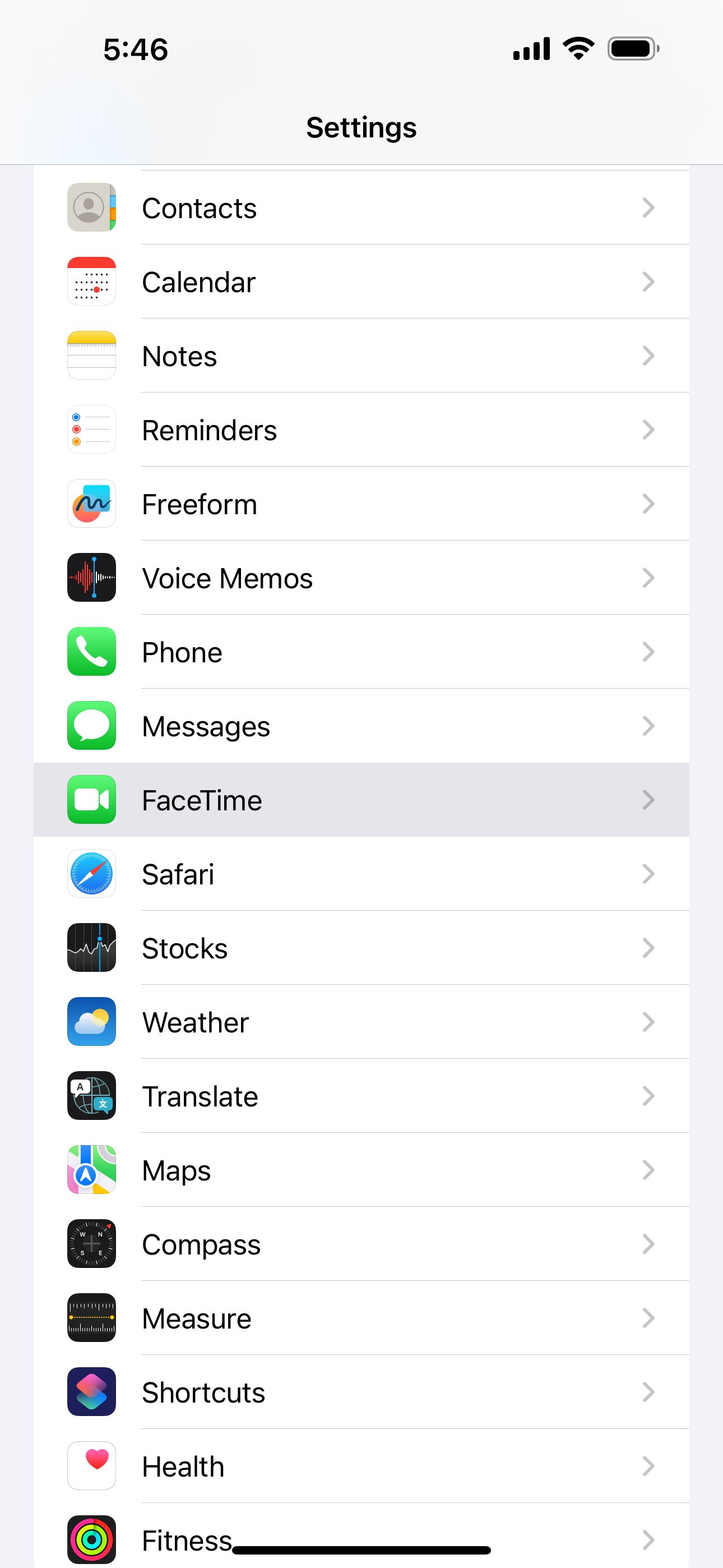The image is a screenshot of a smartphone displaying the 'Settings' menu. The time at the top of the screen is 5:46, and on the right side, indicators show strong connectivity bars and a nearly full battery. The screen lists settings options, each accompanied by an icon on the left, a descriptive word in the middle, and a right-pointing gray 'V' arrow for navigation on the far right.

At the top of the list, the options are: Contacts, Calendar, Notes, Reminders, Freeform, Voice Memos, Phone, Messages, and FaceTime. FaceTime is highlighted in gray, indicating selection, while the other options are white. Continuing down, the options are Safari, Stocks, Weather, Translate, Maps, Compass, Measure, Shortcuts, Health, and Fitness. A short black line appears just below the 'Fitness' option.